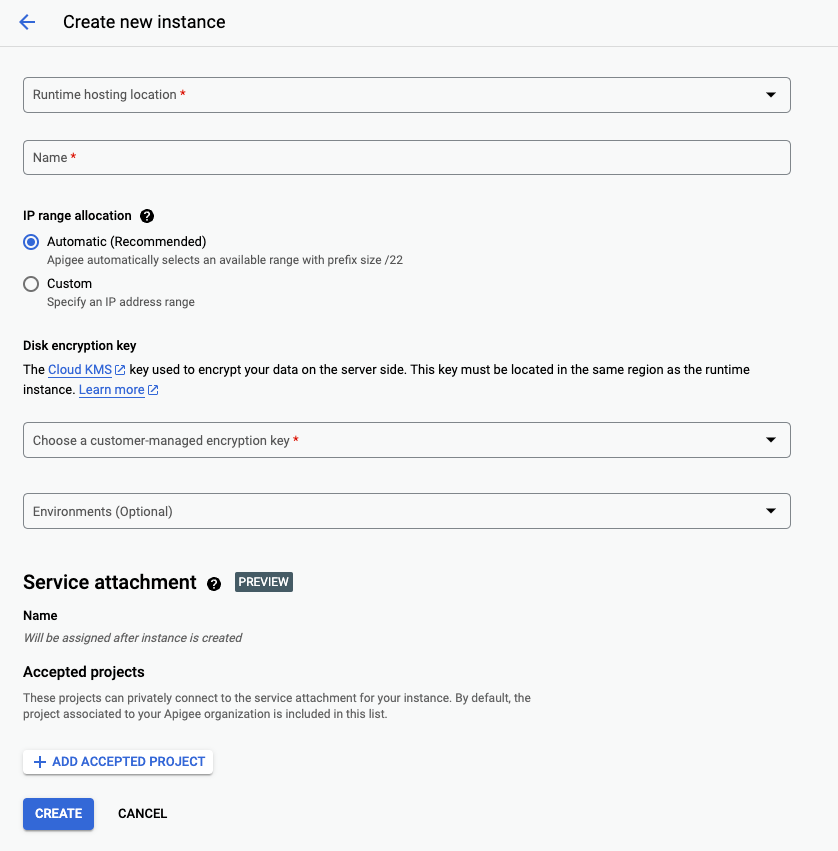### Image Caption:

The image displays a user interface with a grey background and black text. In the top left corner, it features a blue button labeled "Create New Instance." Directly below this button, there are sections for configuring various options:

1. **Runtime Hosting Location**: This is a drop-down menu marked with a red star indicating it is a required field.

2. **Name**: Another required field, also marked with a red star.

3. **IP Range Allocation**: This section offers two options:
   - **Automatic (recommended)**: Automatically selects an available range with a prefix size of 22.
   - **Custom**: Allows the user to specify an IP address range.
   The "Automatic" option is currently selected, indicated by a blue checkmark.

4. **Disk Encryption Key**: Explains that the Cloud KMS key is used for data encryption on the server side and must be located in the same region as the runtime instance. There are two linked texts "Learn more about Cloud KMS" in blue, suggesting additional information is available.

5. **Customer-Managed Encryption Key**: This is a drop-down menu for users to choose a key, indicating that this option is customizable.

6. **Environment**: An optional field for further configuration.

7. **Service Attachment**: Describes that a preview name will be assigned after the instance is created. It also mentions a default project associated with the APG organization, and includes a blue button labeled "Accept a Project" for selection purposes.

At the bottom of the interface are two action buttons:
- **Create**: A blue button to proceed with creating the instance.
- **Cancel**: A black button to abort the operation.